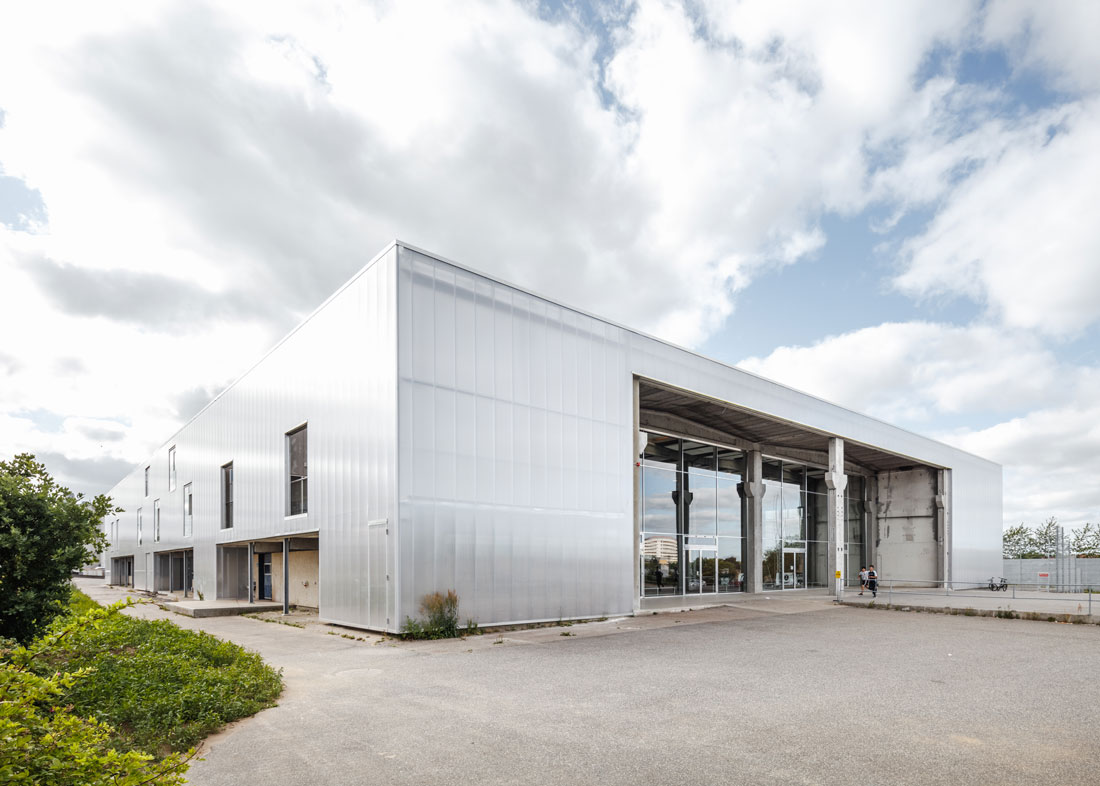This daytime photograph captures a silverish-white, three-story building characterized by its modern design and diverse architecture. The focal point is the building's main entrance, featuring tall, expansive glass windows that reach from the floor to nearly the ceiling, accompanied by two sets of double glass doors. Flanking this impressive facade, two individuals stand, approximately 15 feet from the entrance, near a support pillar adorned with a yellow sign. The building's left side showcases five smaller windows on the second floor, with two additional windows on the third floor. There are hints of bay doors along the bottom, suggesting areas for loading or storage, which is indicative of a possible warehouse or factory function. The environment is partly cloudy with patches of clear sky and the scene is set against a light gray, smooth surface devoid of visible parking lines. The right side of the building is bordered by a fence, while the foreground features a mix of bushes, grass, and a few scattered weeds, adding a touch of greenery to the urban landscape.